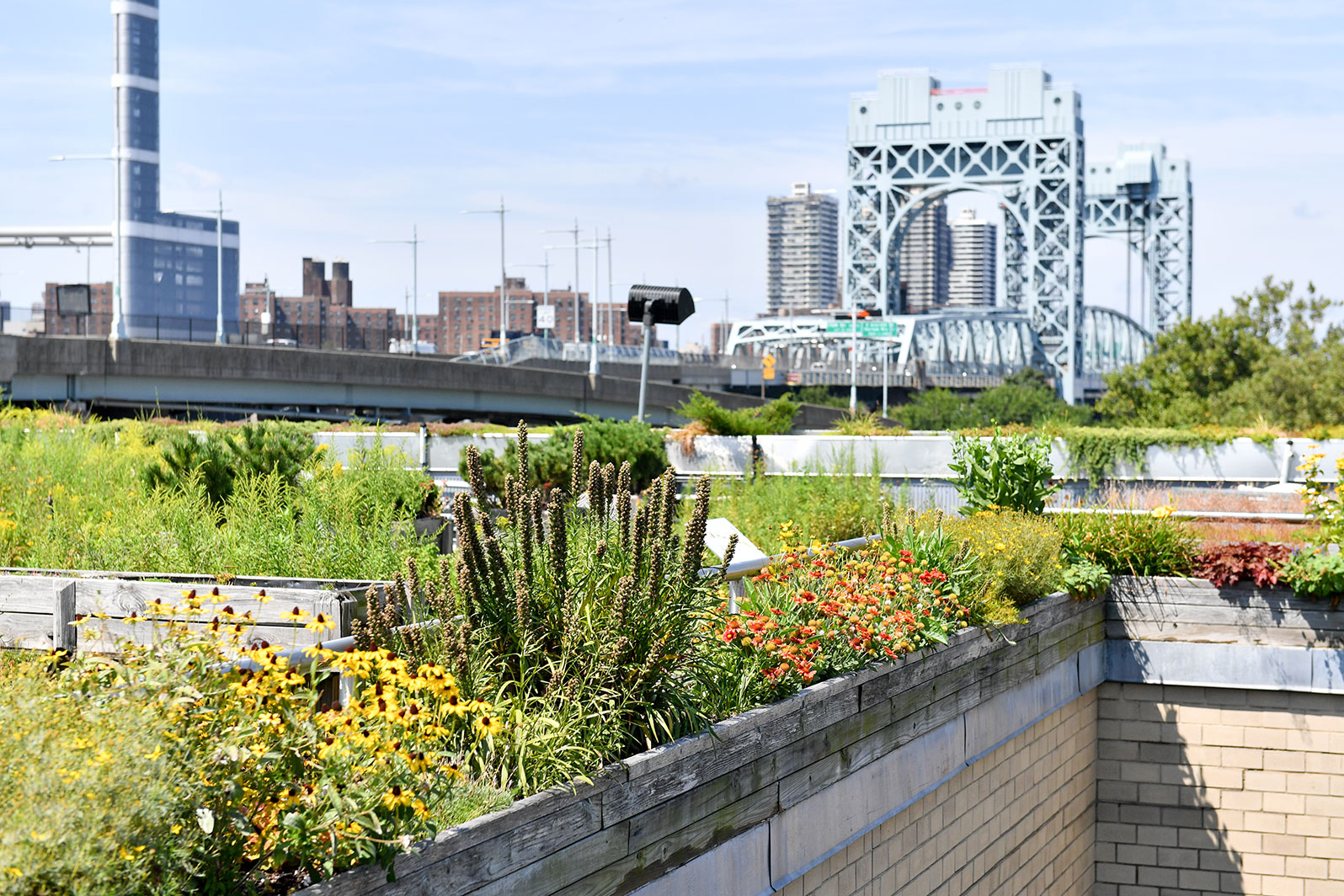The image depicts a vibrant urban garden set against a cityscape backdrop. In the foreground, a wooden planter box sits atop a light brown brick wall, filled with a variety of wildflowers such as cone flowers, Indian paintbrush, cattails, and various greenery, including some bushy reeds. Yellow, red, and purple flowers create a colorful contrast against the rustic planter. The garden appears carefully maintained yet retains a natural aesthetic, possibly functioning as a community space. 

To the left, the garden borders a steep drop-off, reinforcing the need for caution. Behind the garden, the scene transitions to a large, steel bridge with towering arches and light poles lining its sides. This bridge, with its almost light blue hue, stands prominently as a major feature of the urban landscape. 

Beyond the bridge, the city skyline boasts a mix of tall, modern skyscrapers and smaller, older brick buildings. Among these structures is a distinctive L-shaped skyscraper and a tall, radio-shaped glass building. A concrete overpass intersects the image, adding another layer to the urban setting. The bright, photorealistic style of the image emphasizes the juxtaposition of the natural garden against the industrial elements of the city, with the overall setting bathed in the warm, summery light illuminating the mix of yellows, greens, grays, and blues.